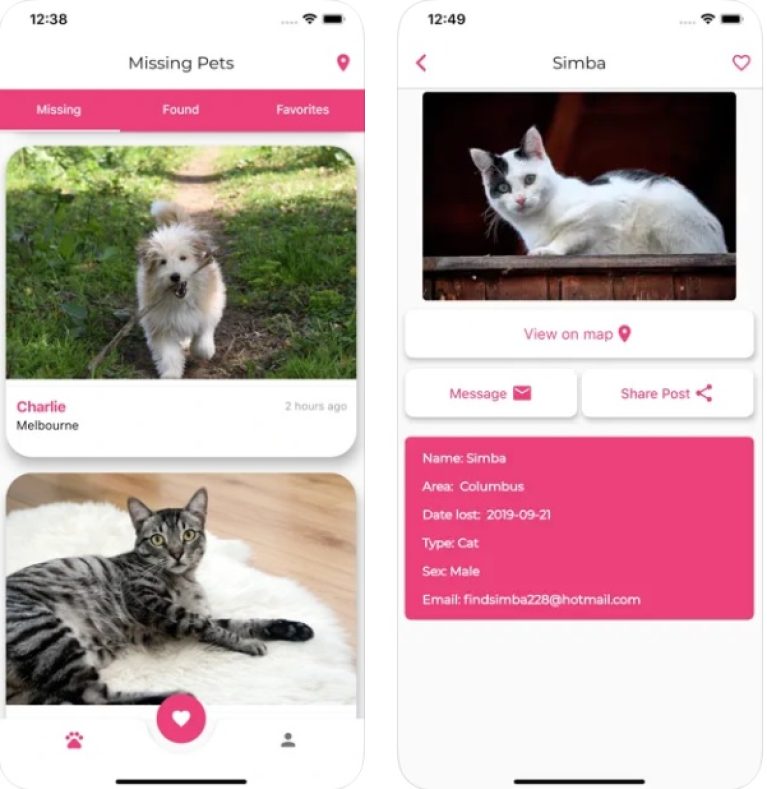The image consists of two separate screen captures from a mobile website dedicated to finding missing pets. Each screen capture features various sections and elements as described below:

### First Screen Capture:
- **Top Section:**
  - **Time:** Displays as 12:38.
  - **Icons:** Wi-Fi signal and battery life indicators.
  
- **Website Header:**
  - **Title:** "Missing Pets" at the top.
  - **Navigation Banner:** A pink banner with options "Missing," "Found," and "Favorites," with "Missing" highlighted.
  
- **Content:**
  - **Photograph:** An image of a furry dog with a stick in its mouth, running on a grassy field. The dog is predominantly white with brown ears, black eyes, and a black snout.
  - **Second Photograph:** An image of a cat inside on a white, bushy rug. The cat has a gray and black mixture of fur and green eyes, looking up toward the photographer.
  
- **Icons and Logos:**
  - Includes a paw print logo, a silhouette of a person, and a central pink circle with a white heart inside it.

### Second Screen Capture:
- **Top Section:**
  - **Time:** Displays as 12:49.
  - **Icons:** Wi-Fi signal and battery life indicators.
  
- **Website Header:**
  - **Title:** "Center Simba," with a left-pointing arrow and a pink heart icon.
  
- **Content:**
  - **Photograph:** An image of a cat sitting on the side of a balcony, predominantly white with black spots.
  - **Buttons:**
    - **View Map:** A white button with "View Map" written in pink.
    - **Message:** A button labeled "Message" to the left.
    - **Share Post:** A button labeled "Share Post" to the right.
  
- **Information Section:**
  - **Background:** A hot pink section with the following details in white text:
    - **Name:** Simba
    - **Area:** Columbus
    - **Date Lost:** 2019-09-21
    - **Type:** Cat
    - **Sex:** Male
    - **Email:** FindSimba228 at Hotmail.com

Each image is laid out on a white background, ensuring the information is clear and the focus remains on the details provided about the missing pets.